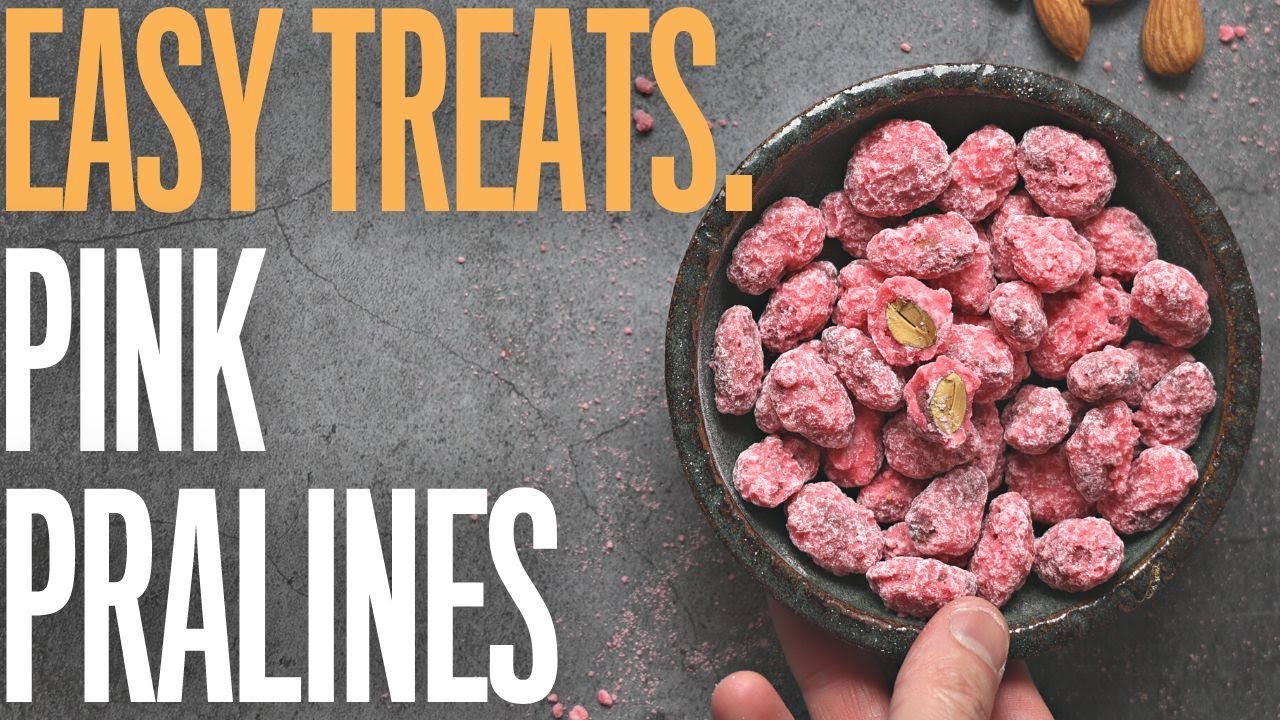The image features an appealing advertisement for pink pralines. On the left side, in large orange text, is the bold caption: "Easy Treats," followed by "pink pralines" in white text. On the right, a polished stone bowl, potentially held by a man's hand, displays a collection of the pink pralines. These pralines are coated in a sugary, frosted pink substance with a white dusting, giving them a candied appearance. The bowl contains some whole pralines while two are halved, revealing their nutty centers. In the top right corner of the image, a few raw almonds can be seen, providing a contrast to the sugary treats. The overall setting of the image is unclear, possibly inside or outside, but it clearly emphasizes the delectable appearance of the pralines.